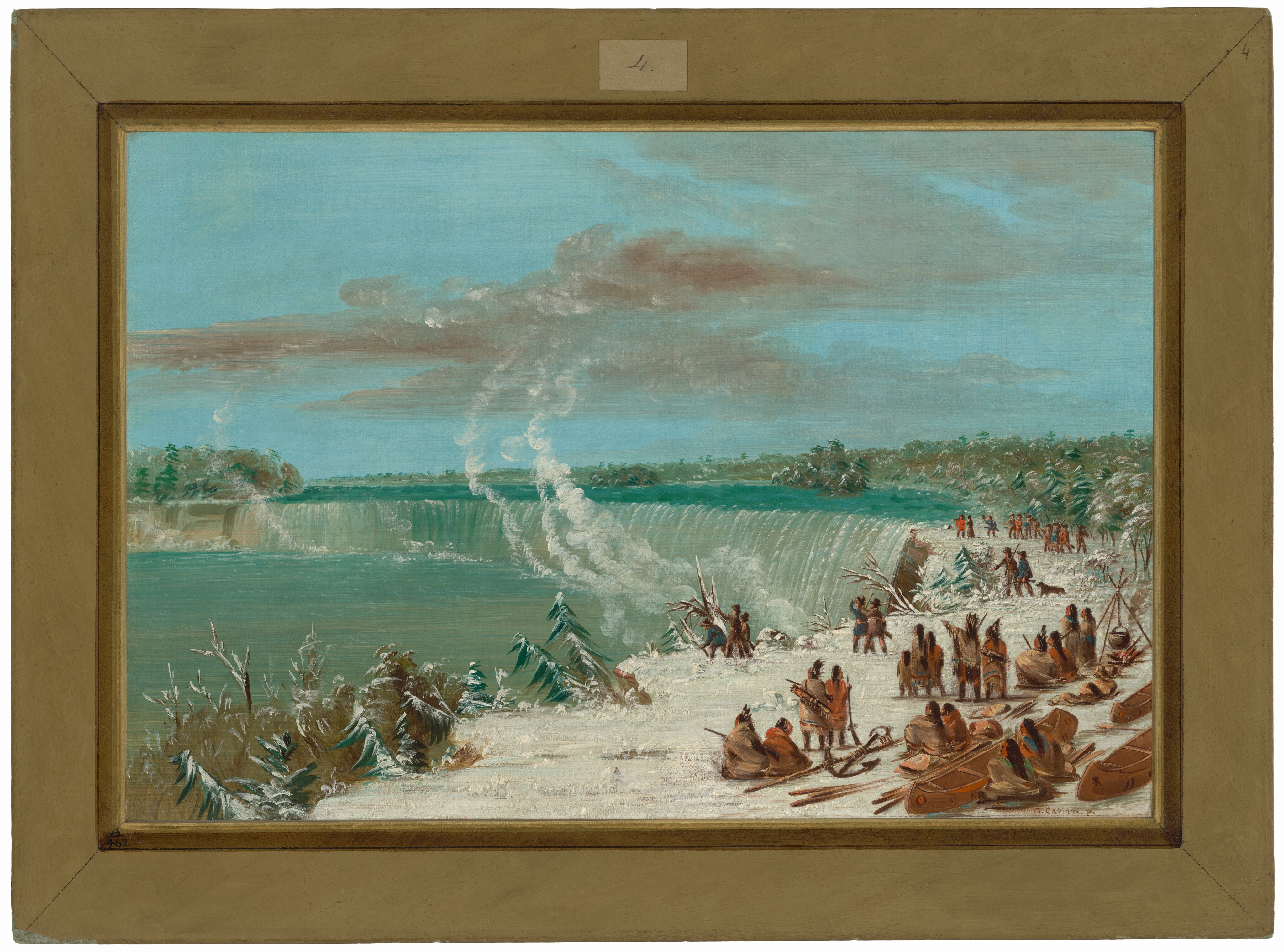The painting is framed in a brown frame and presents a detailed scene featuring Native Americans interacting with their environment. Dominating the left side of the canvas, a stunning waterfall with sea green waters cascades down into whiter falls, emitting what appears to be smoke or mist. On the right side, a ground area covered in what looks like snow—though, it might be sand—hosts numerous Native Americans engaged in various activities. They are depicted with brown clothing and some are wrapped in blankets. The people appear to be families and small groups, including children, mingling, chatting, and working on canoes placed on the ground. Surrounding the scene, lush vegetation, including pine trees dusted with snow, extends into the distant horizon, blending into the azure blue sky dotted with brown clouds. The overall setting gives an impression of everyday life amid nature's stunning beauty, with a harmonious balance of water, ground, and sky.